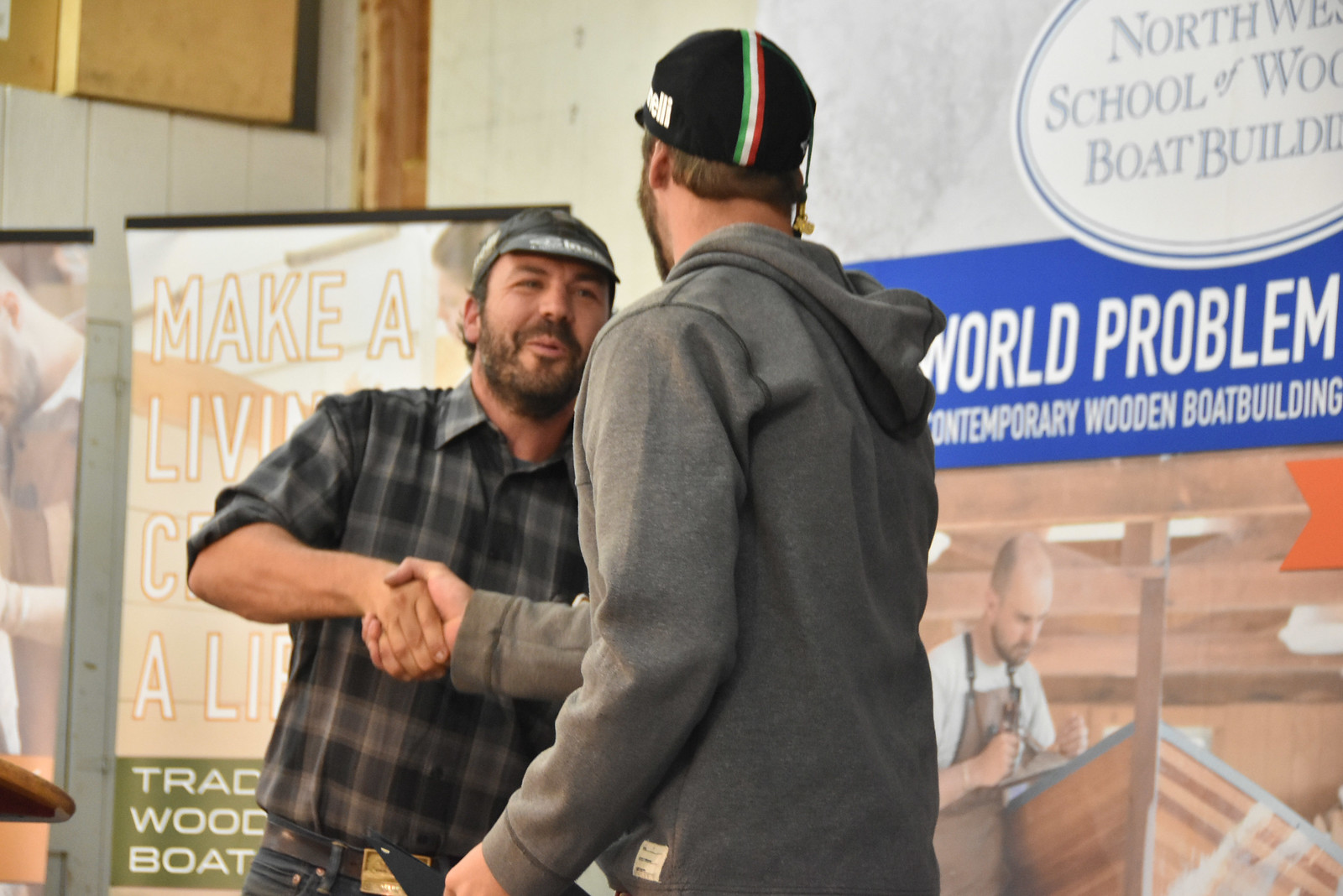In this outdoor photograph, two white men are shaking hands, standing in front of several signs. The man on the left is facing the camera, wearing a dark hat with a very narrow bill, a gray and black button-down collar shirt in a plaid pattern, blue jeans, and a belt. He has short brown hair, a brown beard, and a brown mustache. The man on the right, facing away from the camera, is dressed in a gray hoodie and a black hat adorned with a green, white, and red stripe down the center. Behind them on the wall is a large off-white sign with a blue border that reads, "Northwest School of Wood and Boat Building" and "Contemporary Wooden Boat Building." To the left of this main sign, there are additional signs, one of which prominently features the phrase "Make a Living." The background suggests they are at a boat-making class or event, and a photo of a man building a boat is depicted on one of the signs.